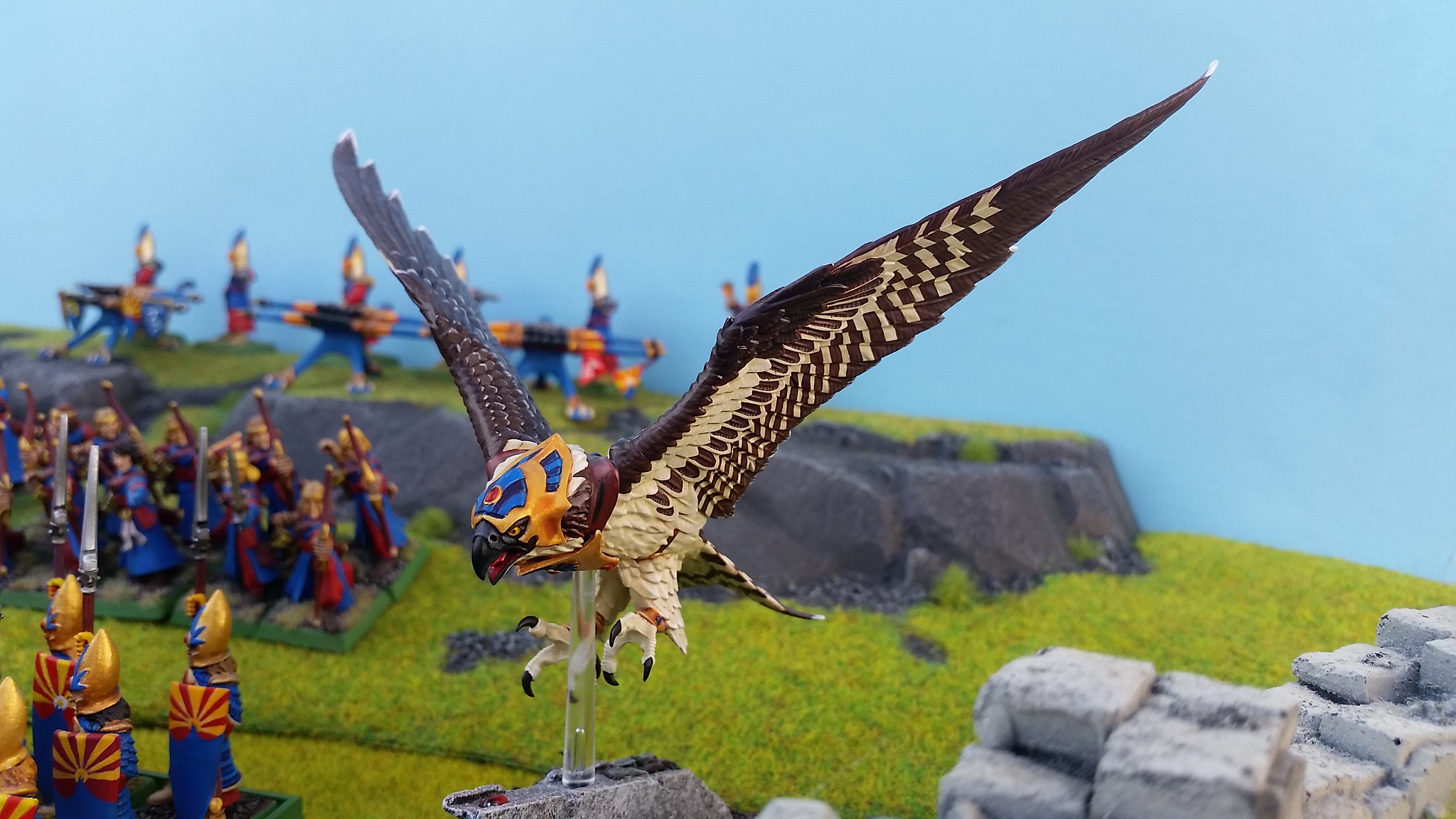The image depicts an intricate miniature battlefield diorama, evocative of an Asian fantasy or historic scene. The centerpiece is a majestic giant falcon with outstretched wings, poised in mid-swoop with its talons extended towards the ground. The falcon is adorned with an elaborate, gold helmet featuring blue and purple streaks, and a prominent red gem set in its forehead, exuding an almost Egyptian aesthetic. The bird itself displays a striking coloration, with a predominantly white body and brown wings, while its feet are white with black talons. It is attached to a clear, plastic stand that gives the illusion of flight above the terrain.

The battlefield is rendered on a textured surface resembling green-yellow felt or peat moss, adding to the realism of the scene. In the foreground are infantrymen equipped with distinctive rectangular shields bearing a sunburst design – the upper third radiates red and yellow, reminiscent of the Japanese flag, while the lower two-thirds are blue. These soldiers also wear gold helmets with blue accents and a similar red dot in the center, tapering to a pointed top.

Further back, additional infantry units can be seen, including archers with bows ready and lines of soldiers possibly managing ballistae or mounted guns, all maintaining the striking red, blue, and gold color scheme. On a rocky ridge, figures are depicted holding long poles, suggesting a method of transporting royalty. The scene is bordered on the right by a formation of gray-white square stones arranged like a wall, while the backdrop consists of a blue surface that could either represent the sky or a painted background wall.